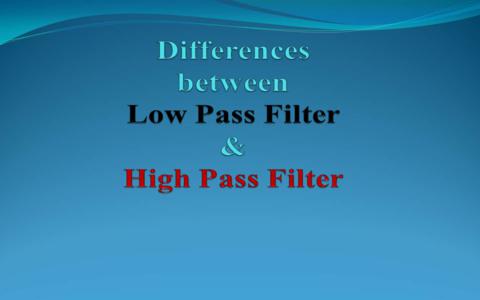In this informational image, we see a detailed comparison between a low-pass filter and a high-pass filter. Dominantly blue in theme, the top section features a series of wavy lines with light blue and dark blue hues creating a water-like effect. The text "Differences Between" is prominently displayed in light blue at the top. Beneath, "Low Pass Filter" is written in black, followed by an ampersand in light blue, and "High Pass Filter" in red. The bottom part of the image continues the blue background, which adds a cohesive look to the informational card or poster. This color contrast and wave design enhance the visibility and differentiate the types of filters being discussed.